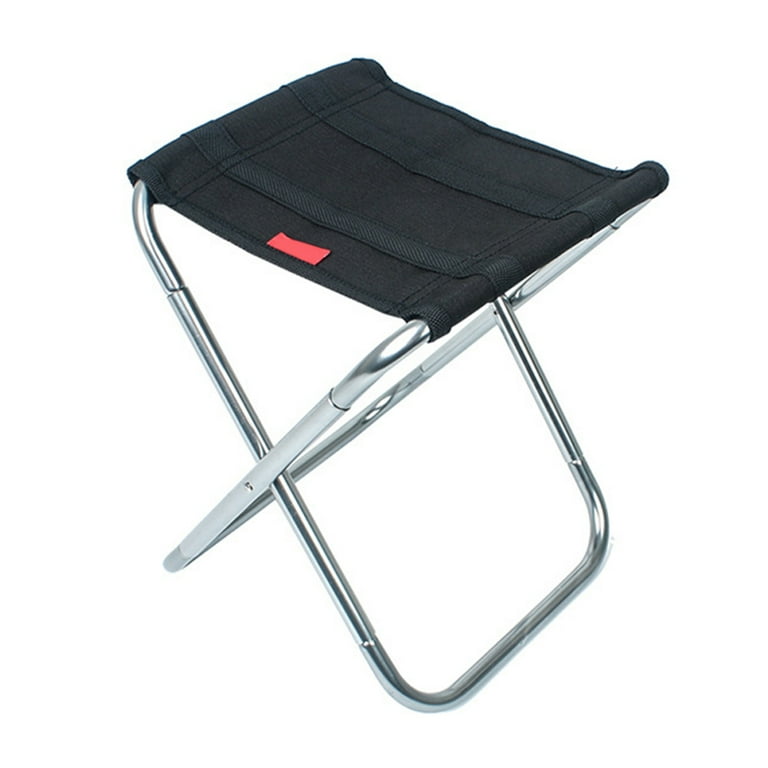The photograph features a collapsible camping stool set against a white background. The stool is designed with a sturdy, X-shaped metal frame, likely made of aluminum or stainless steel, which provides a stable base when unfolded. The seat is constructed from black nylon fabric, which is both durable and comfortable, with the fabric sewn securely around the frame. A distinct red label is located on the front of the seat. Compact and portable, the stool can easily be folded for storage or transport, making it ideal for camping trips or outdoor activities.